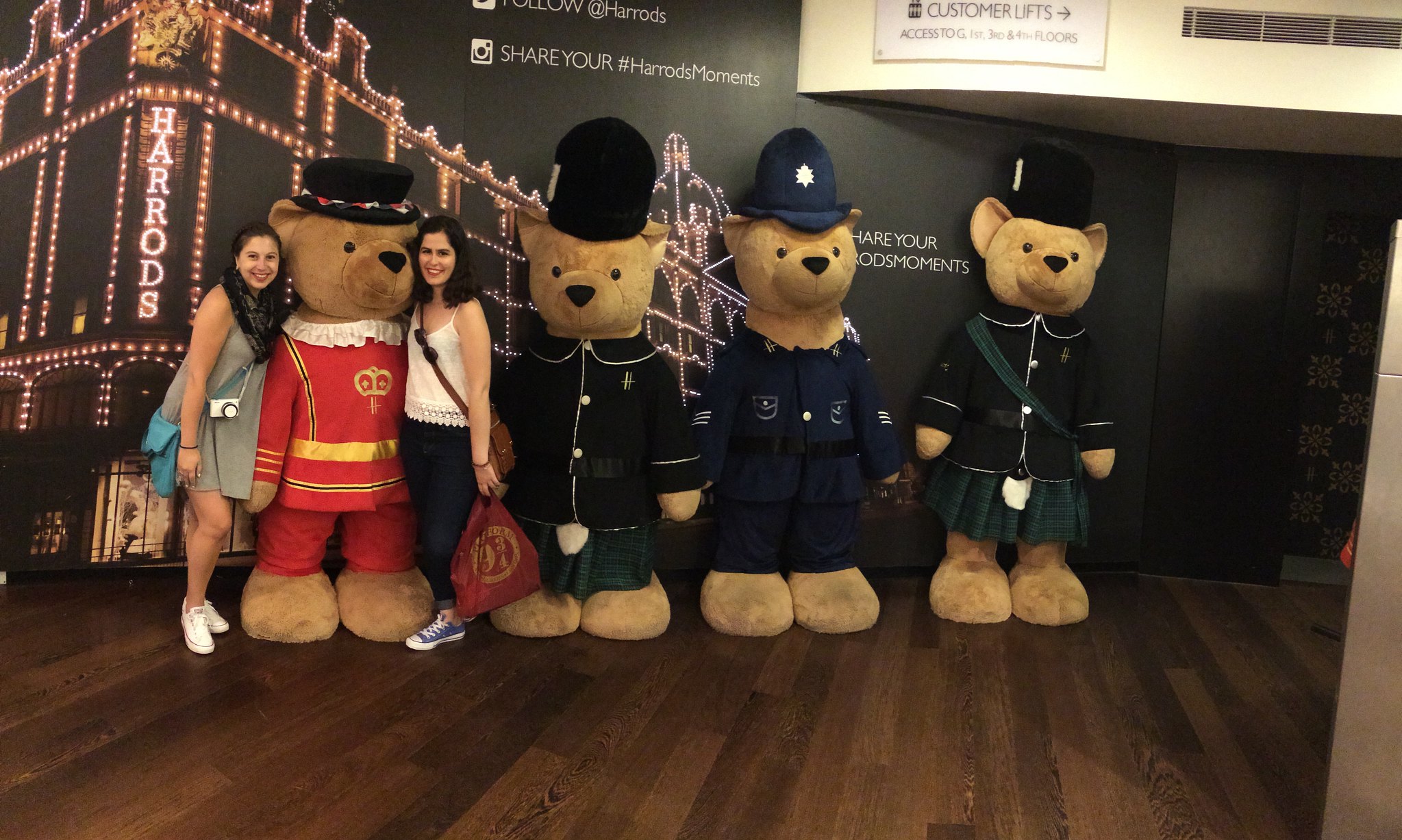The image depicts a set of four human-sized teddy bears on display at Harrods, a renowned department store in London. Each bear is dressed in a distinct, elaborate outfit and stands tall with characteristic features such as big puffy feet, black eyes, and a prominent black nose. The bear on the far left is adorned in a striking red suit embellished with gold accents and a crown motif, complete with a white ruffled neckline. This bear has a shallow hat perched on its head and is accompanied by two young women posing for a picture, indicating they might be tourists, as they are holding cameras and shopping bags. One woman is dressed in a teal-colored dress with a blue handbag and white shoes while the other sports a white top, black pants, and carries a maroon bag.

The second bear from the left is outfitted in a classic black coat paired with a green kilt and topped with a bulbous hat, giving it a distinguished appearance. Next to it is a bear in a policeman's uniform, featuring a navy blue color scheme. The bear on the far right wears an ensemble similar to the second bear but with the addition of a green sash crossing its chest, highlighting its green-based attire.

In the backdrop, there's a large printed advertisement sign proclaiming "Harrods," further situating the scene within this iconic London store. The backdrop includes additional text and imagery that enhance the promotional setting. The entire display creates an inviting and whimsical scene capturing the attention of passersby and inviting them into the magical world of Harrods.